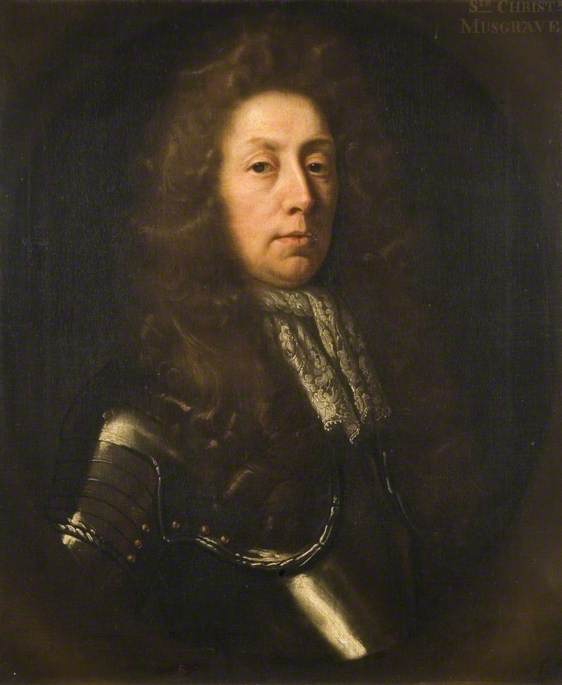This is a portrait oil painting of Sir Christopher Musgrave, created by artist John Riley, who was active in the mid to late 1600s. The composition focuses intensely on Sir Christopher's upper body against a completely black background, bringing significant emphasis to his face. The portrait captures him just above the waist up, with his face slightly tilted, offering a partial profile view. Sir Christopher, a white man appearing to be in his 50s, has long, dark brown hair that blends into the dark background and his equally dark attire. He wears a gray-silver scarf tied just below his neck, draping over his jacket, adding a touch of distinction to his otherwise sober clothing. His expression is serious, almost solemn, with pursed lips and piercing eyes that stare directly out towards the viewer, betraying no emotion. The stark contrast between his illuminated face and the dark surroundings highlights the intensity of his gaze and the refined details of his distinguished features.